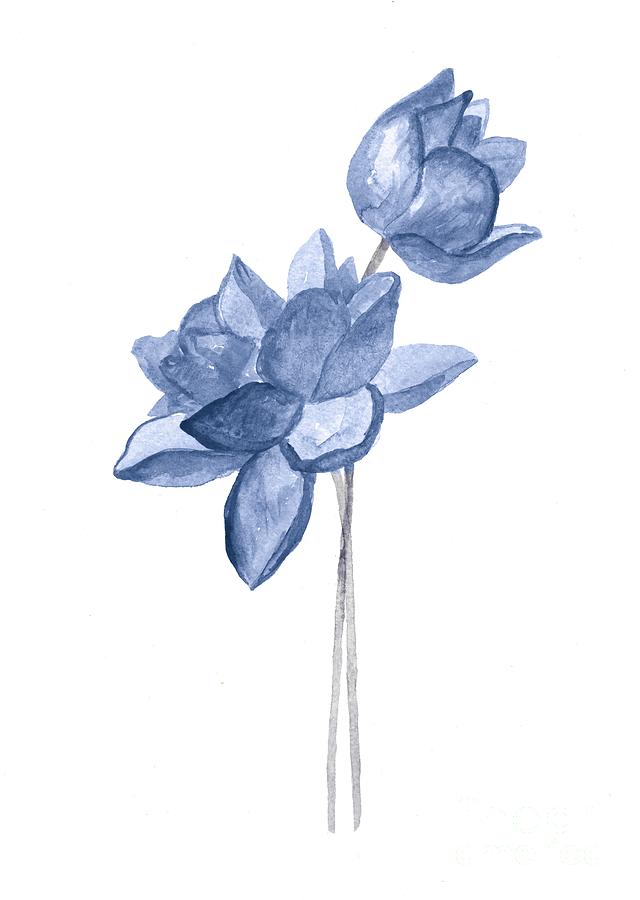This is an intricate hand-drawn watercolor painting of two blue lotus-like flowers on tall, thin stems set against a completely white background. The stems, starting at the bottom, transition from light gray to dark gray as they rise. The flower on the left is more open, featuring light blue petals with darker edges and a couple of darker petals in the center, giving it a vibrant appearance. Its petals are spread apart, showcasing a layered bloom with the lower ones lying flat and the upper layers cupped and pointing upward. The flower on the right, which is taller and more closed, has a rounded bottom and features a dark blue petal with a white blotch at the top and dark blue lines along the petal edges. Both flowers exhibit a range of blue shades, from light to dark, emphasized by white highlights that add a realistic touch. The overall composition gives a harmonious yet dynamic visual of two flowers at different stages of blooming, with the front flower fully opened and the rear flower just beginning to bloom.